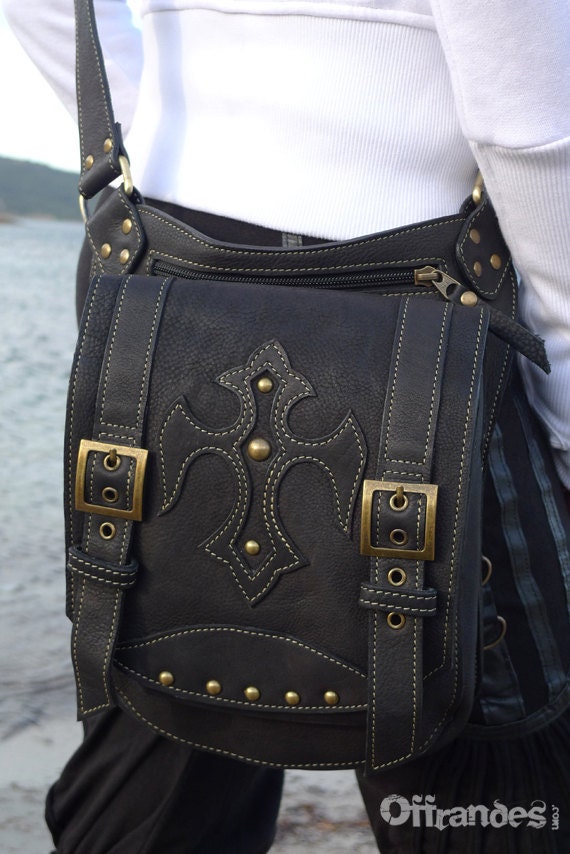The photograph, oriented in a portrait layout, prominently features a meticulously crafted black suede leather backpack, adorned with intricate details. The focal point of the image is this rectangular-shaped bag, which boasts gold stitching and brass hardware. The long strap of the backpack crosses over a person's body, situating the bag against their backside, effectively covering their behind. 

The backpack showcases a blend of aesthetic and functional elements, including brass rivets along the strap and eyelets on a side pocket flap, which is secured with a brass buckle. Additionally, it features a stylized cross pattern, reminiscent of a fleur-de-lis, centered with three brass studs—one large in the middle and two smaller ones above and below. The bag's edges are finely sewn with white thread, which might be machine stitched or hand-sewn, adding to its detailed craftsmanship.

The individual wearing the backpack is dressed in a white cotton shirt with segmented stitching details along the sleeves and chest, paired with black pants that appear slightly slack. In the background, the setting offers subtle hints of a natural landscape—a possibly gray, fine soil or rocky ground beneath and a mix of white sky and distant greenery, perhaps suggestive of a beach or lakeside environment. The image also displays the text "Offrandes" in the bottom right corner, which may indicate the designer or brand of the beautifully detailed backpack.